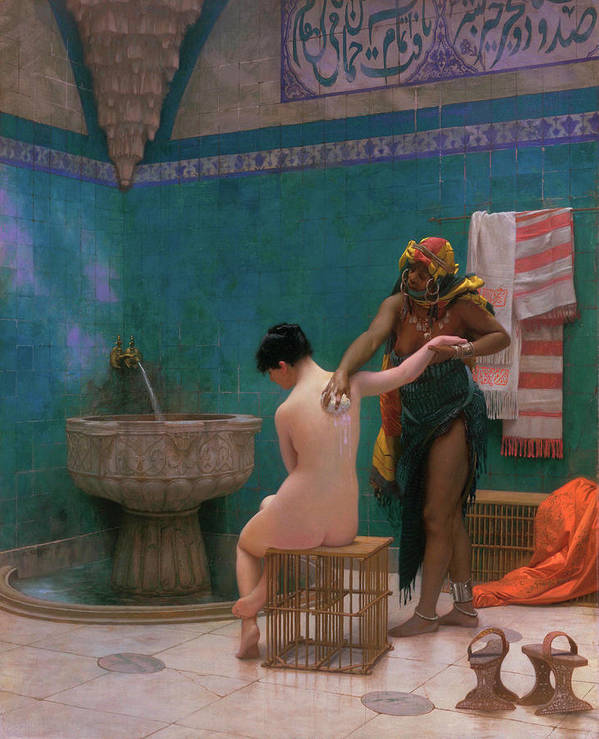The painting depicts an intimate scene in an old-time bathhouse. At the center, a naked white woman sits on a wooden, cage-like platform, her back turned towards the viewer, looking down at the floor. She is being gently washed by a darker-skinned individual wearing a vibrant yellow and red headdress and a dark green wrap around their waist. The imagery captures water flowing from a fixture built into the turquoise blue-tiled wall, cascading down into a stone basin below, evoking the image of a fountain. Hieroglyphic-like inscriptions adorn the upper part of the wall, adding an air of mystique. To the right of the composition, an orange robe or sheet drapes over another platform, accompanied by red and white striped towels hanging on the marbled wall. The entire setting is framed in a teal and tan-colored bathhouse, conveying a sense of historical and cultural richness.